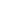In this lively street scene on a cloudy day, a female mime captivatingly stands out amidst what appears to be a bustling fair or festival. Dressed in classic mime attire, she dons a black beret adorned with a black and white striped bow. Her face is strikingly painted white, with pronounced black eyebrows, delicate pink accents beneath them, and bright red lips. Black dots and eyeshadow further embellish her expression. She wears a black and white striped shirt, complemented by a black skirt, with blue ribbons attached to her shoulders and white gloves on her hands. A vibrant red rose is pinned near her chest, adding a touch of color.

The mime is poised with her head slightly tilted to the left and her shoulders slightly to the right, while she blows a kiss towards the camera, her flesh-colored neck visible above her costume. In the background, a group of onlookers stands to the left, watching her performance with interest. To the right of the image, a red-haired woman clad in a black shirt and skirt is positioned next to a stall. The stall features a white canopy, a blue backdrop, and a blue tablecloth, suggesting an inviting atmosphere of the ongoing event.